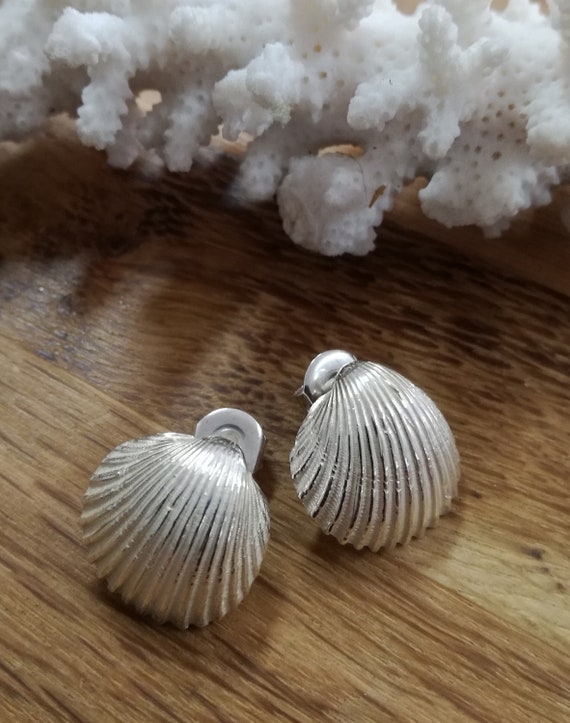The photograph captures an indoor scene featuring a white coral or calcite centerpiece resting on a brown wooden table. Below the coral, a pair of seashell earrings are prominently displayed. The earrings, shaped like cockle or clam shells, have a silver hue with intricate black lines accentuating the grooves of the shells. They culminate in metallic clasps, either silver or gray, that could indicate they are either clip-on or stud earrings. The table is otherwise bare, emphasizing the detailed textures and colors of both the coral and the earrings.